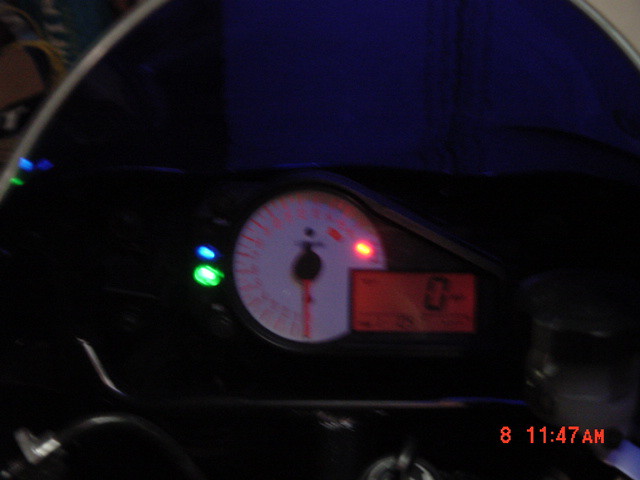In this dimly lit and blurry image, the focal point is a speedometer, which appears somewhat out of focus. The speedometer itself is distinct with a white face, during illuminated with backlit orange lighting. The needle, which is also orange, is prominently visible despite the blur, though the exact numbers on the gauge are indiscernible. Surrounding this central gauge are a few other illuminated lights in various colors – green, blue, and red – contributing to the overall glowing effect.

Next to the speedometer, there is an illuminated rectangular digital display that shows the number zero against an orange backdrop. This likely serves as a supplemental speed readout, indicating either kilometers or miles per hour. The context of the image suggests that the speedometer is connected to some power source, evident from the illumination, but it remains unclear if it is mounted within a vehicle or attached to another setup, possibly for testing or monitoring purposes.

The background of the image remains largely in shadow, with vague outlines hinting at possible dashboard elements in black, along with an indistinct blue and white component. Overall, the image conveys a sense of an active, illuminated instrument panel, surrounded by darkness and blur, making detailed assessment challenging.